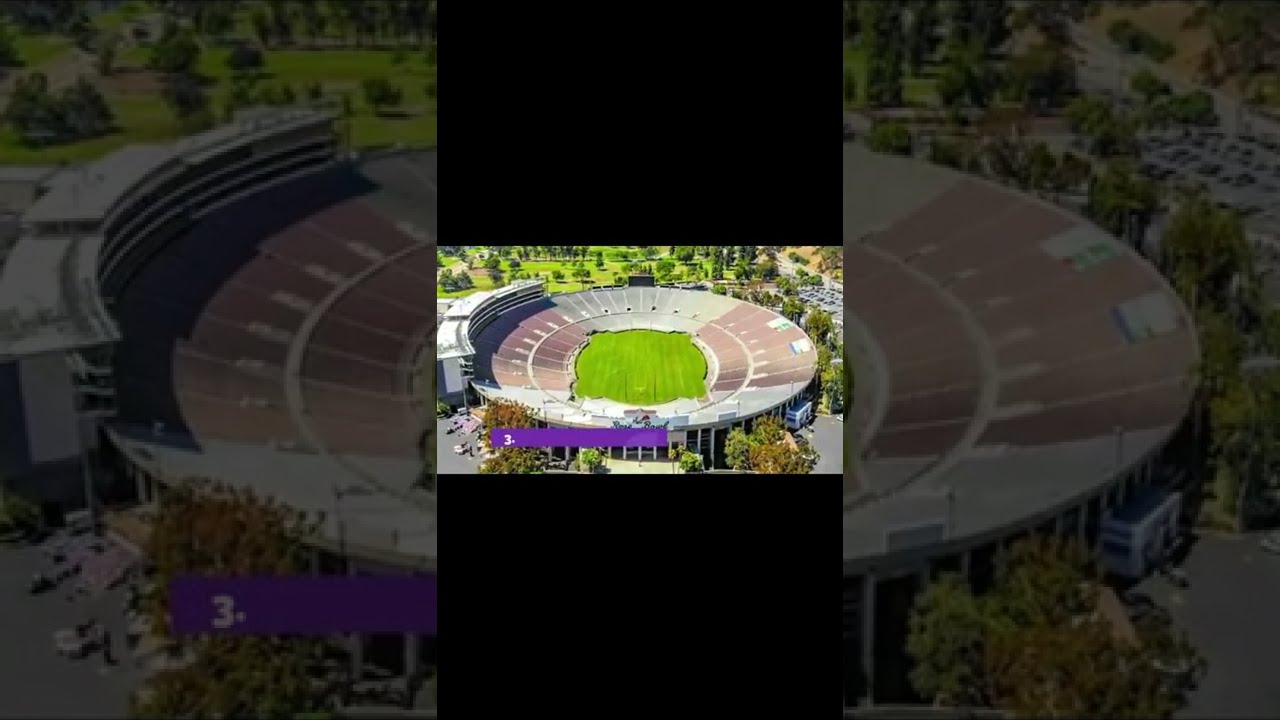The image is divided into three vertical sections, with the middle section displaying an aerial view of an oval-shaped stadium. The stadium features a bright green field in its circular center, surrounded by seats that are primarily red and green. Above and below this central part, there are horizontal black bars, which further frame the image. The left and right thirds of the image are darkened close-ups of the stadium's left and right sides, respectively. These enlarged sections highlight the stadium's detailed structure, including portions of a purple banner at the bottom edge with a white number three on the left side. The stadium has a mix of brown and gray seats, with an extra tall building-like attachment on the left side, characterized by black windows at the bottom and white stairs on the exterior. Surrounding the stadium, one can observe gardens, parking spaces, and several trees, particularly prominent at the top and right side of the stadium. Near the top-right corner, there is another grayish building with an orange rooftop.